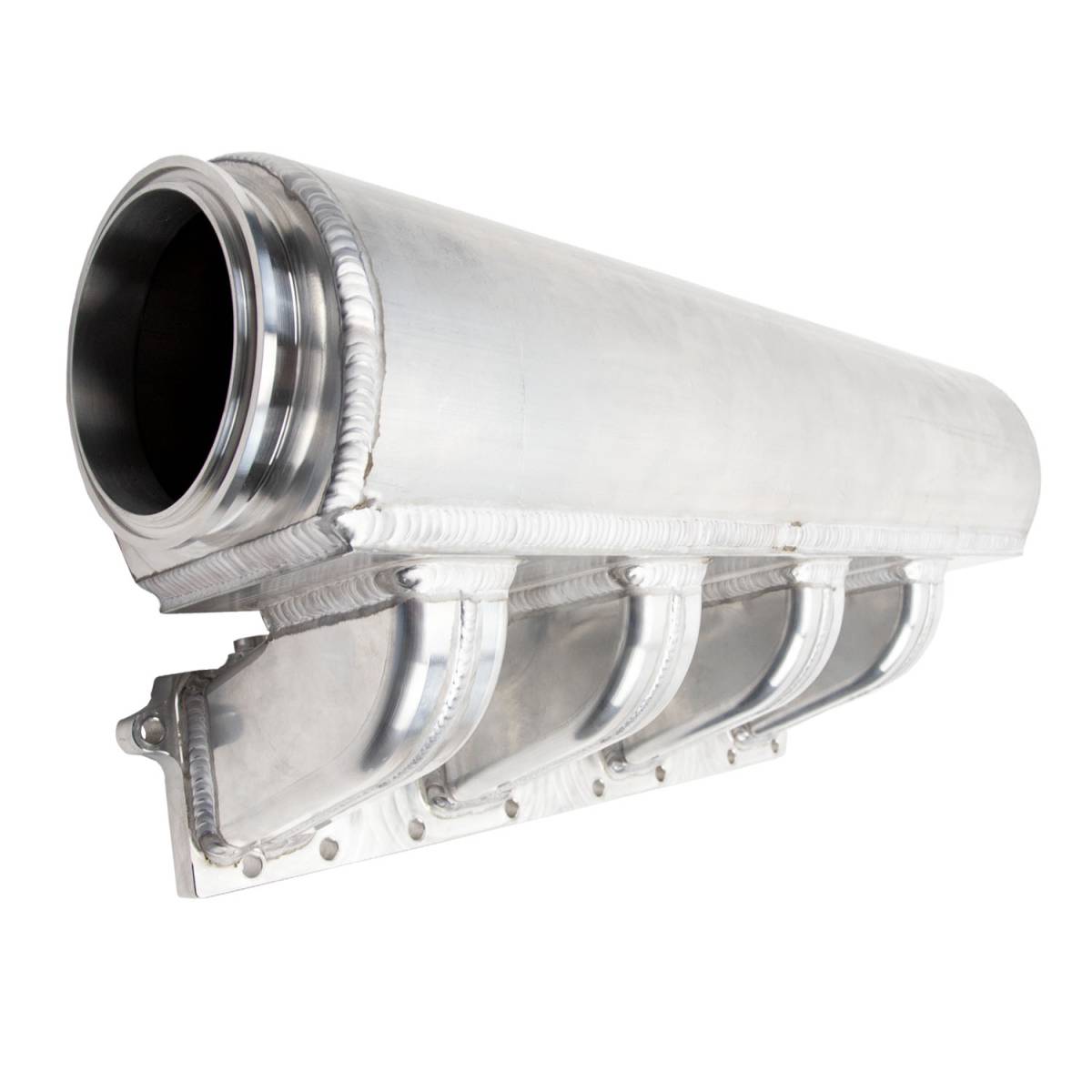This image features a silver-colored metallic tubular structure, possibly part of an engine block or car exhaust system. The photo is taken from an angle, slightly tilting the front end towards the camera with the right end appearing more distant. The main body of the cylindrical tube stretches horizontally from left to right. On the left end of the tube, a rim is visible, and just inside, it appears black. Sturdy metal fixtures are attached to the bottom of the tube; there are four, each curving back toward the left, creating an intricate and aesthetically pleasing welded pattern. These fixtures connect to a base featuring screw holes, suggesting they are meant for secure attachment, likely onto a vehicle or mechanical component. The photo is set against a neutral, likely transparent or white background, providing a clear view of the detailed metalwork and the sophisticated craftsmanship in the welding and assembly of the tube and its components.